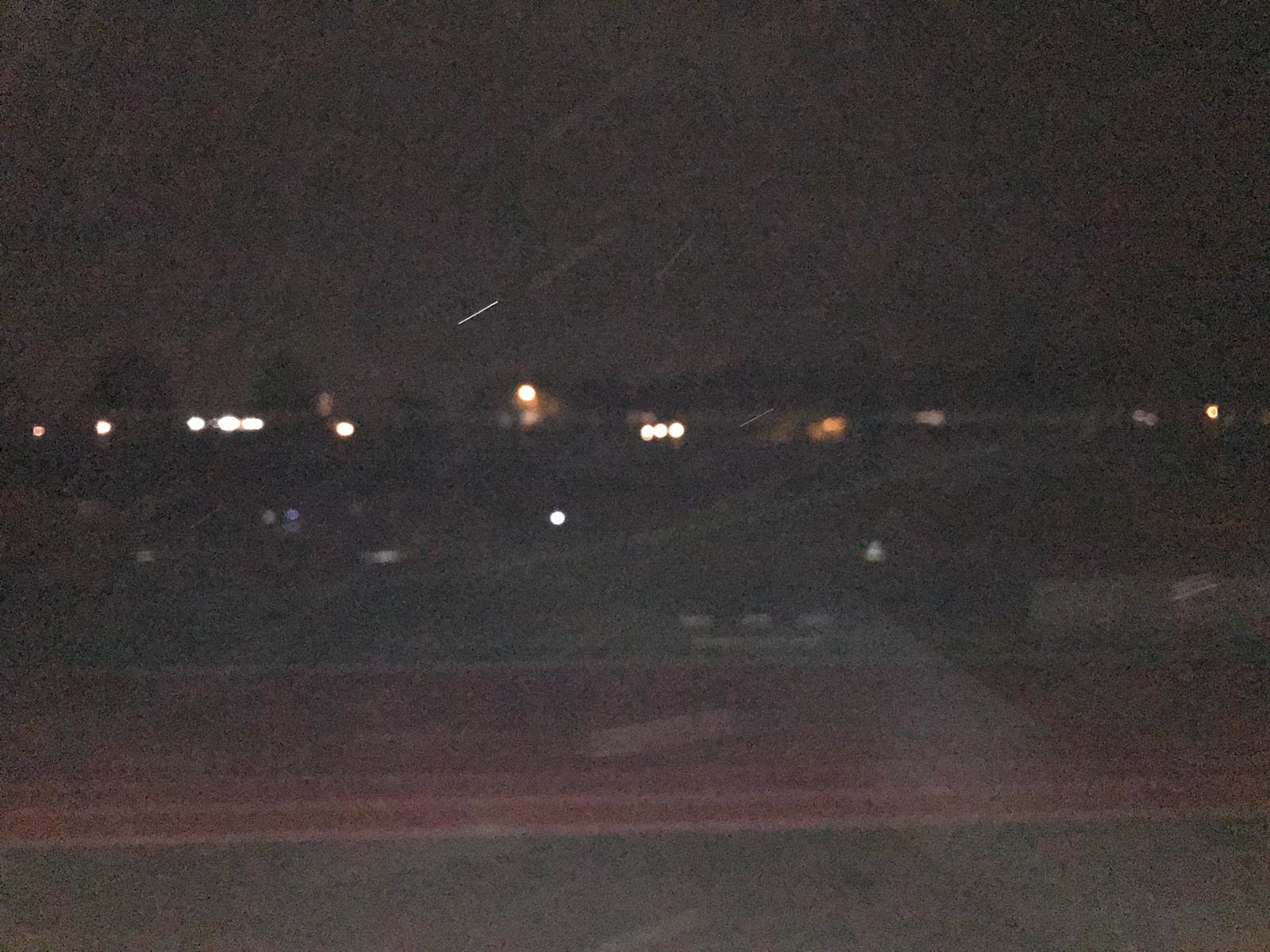A blurry, nighttime photograph captures an outdoor scene, giving it an unfocused, almost abstract quality. Rainfall blends with the camera’s poor focus to create a chalky white effect, adding to the moody atmosphere. The image appears to have been taken near a running track, indicated by the red and white ground markings. In the background, distant houses are discernible, their presence hinted at by clusters of lights that range from grouped to solitary, mimicking the glow of porch lights piercing through the gloom.